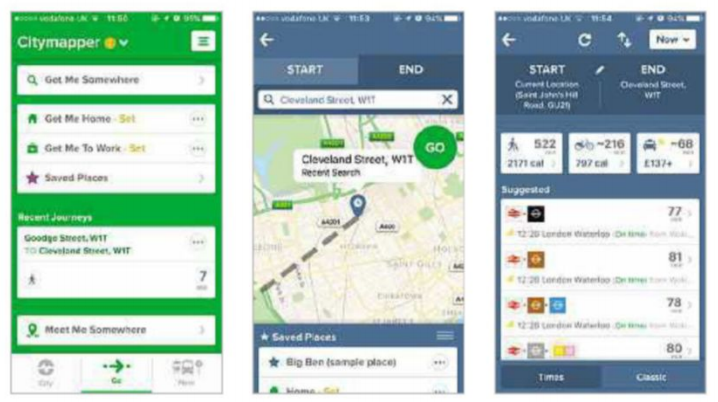This image is comprised of three slightly pixelated screenshots that showcase a navigation app interface. Each screenshot displays an organized layout of features, icons, and options within the app.

The first screenshot has a predominantly green and white background. At the top, familiar interface icons are visible, including the cell phone carrier signal, Wi-Fi icon, time, and battery percentage. Below this, the screen is primarily green with a large "Citymapper" title and a gold circle. It includes green and white boxes for options such as "Get me somewhere," "Get me home" with a house icon, and "Get me to work" with a briefcase icon. Below these, a purple star icon labeled "Saved places" is shown, followed by an address labeled "Good day street" in green. The screenshot also features a "Meet me somewhere" option marked with a green location pin. At the bottom, grey navigation icons include a green arrow and a grey bus.

The second screenshot has a blue and white background. It begins with a back arrow and options labeled "Start" and "End," along with a magnifying glass icon for searching. It displays the name "Cleveland Street," along with a map view in shades of grey, green, and tan. Additional elements include "Recent search" and a "Go" button in a green circle. There are also "Saved places" marked with a blue star and another green circle.

In the third screenshot, the top portion again features "Start" and an address marked as "End" in white text. Below this, several boxes display icons and caloric values: a person icon indicates 522-2171 calories, a bike icon shows 216-797 calories, and a car icon lists 68-137 calories. A "Suggested" label is followed by white boxes containing black, red, gold, and blue icons and corresponding black text with numbers such as 77, 81, and 7880. Finally, two additional blue boxes are present near the bottom.

These screenshots collectively highlight various navigation and search functionalities, as well as saved and suggested routes, within the navigation app.